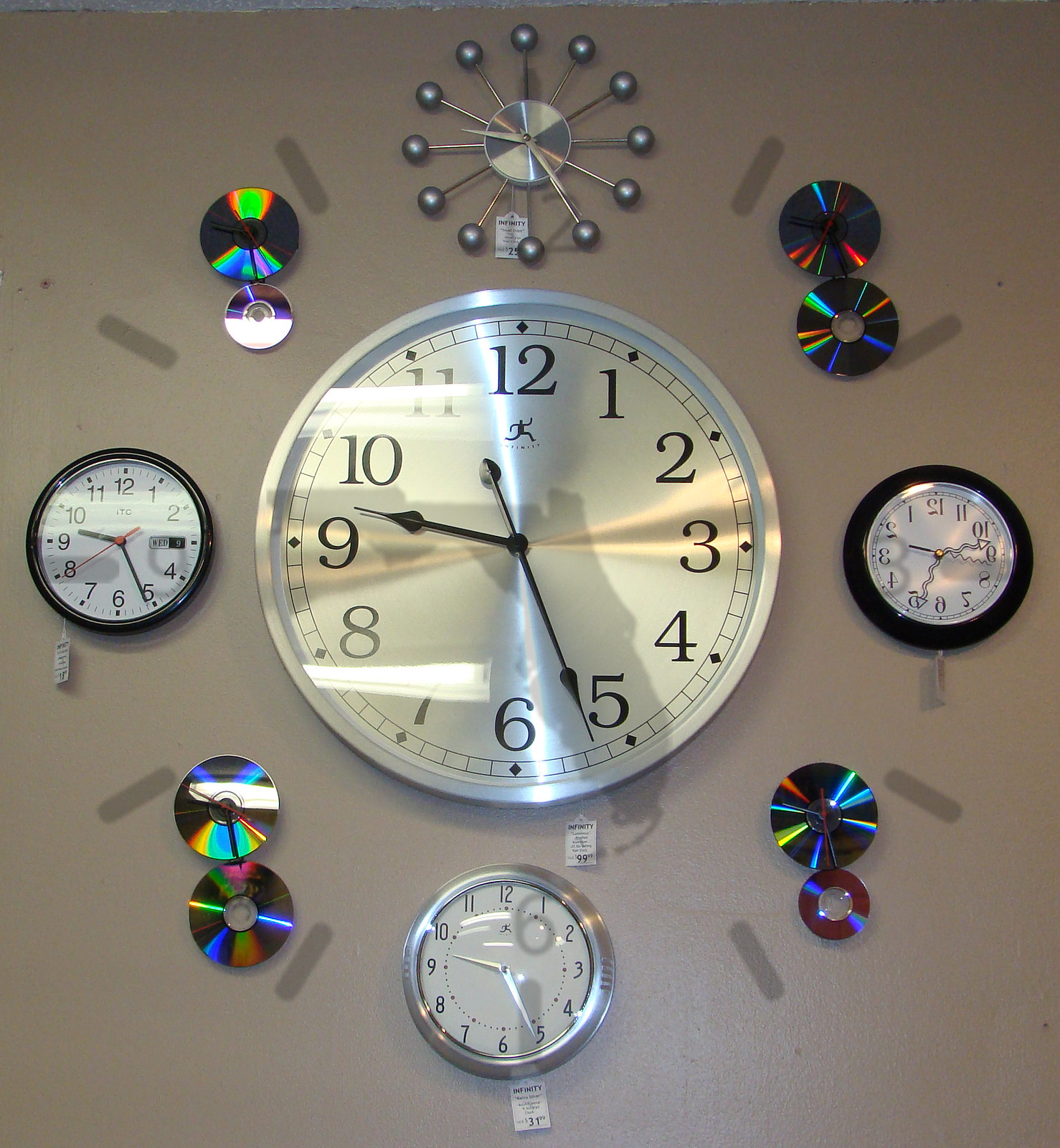A square image shows a downward view of a surface, either a brown table or a wall, adorned with several clocks arranged in a symmetrical pattern. The centerpiece is a large silver clock with a white face featuring black numeric numbers, displaying the time as 9:26. Below it sits a smaller silver clock, also with a white face and numeric numbers. Flanking the central clock to the left and right are two smaller black clocks, both devoid of Roman numerals. Adding a decorative touch, each corner of the image features shiny silver discs that reflect light, creating a prism-like effect.